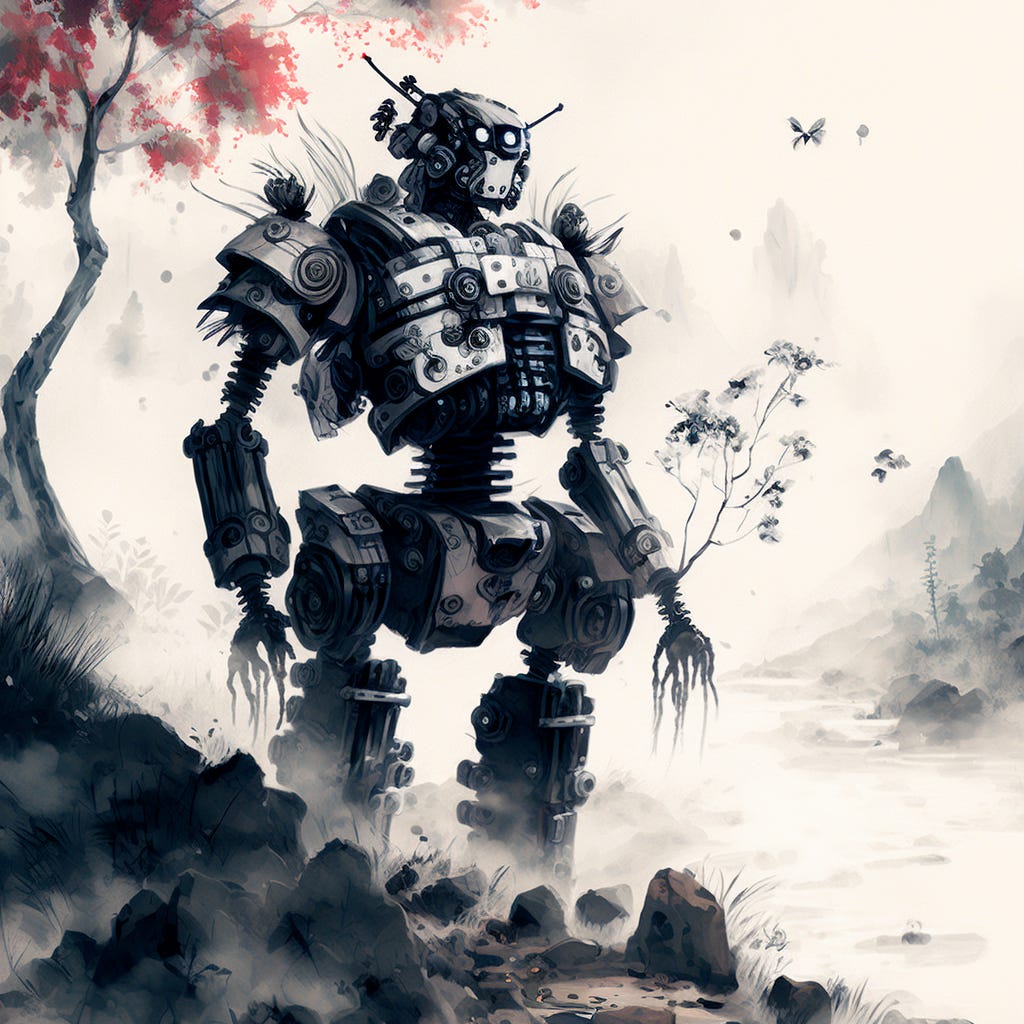The digital artwork depicts a large robot standing in the center of the image. The robot is constructed from various metal components, featuring silver and black hues with screw-shaped parts in its arms and torso, and fingers resembling tree roots. Its design includes circular parts integrated into its body. The background is primarily white, allowing the grayscale elements to stand out. To the left of the robot, there is a small, seemingly buried mountain, surrounded by rocks in shades of gray and black. A tree with striking red leaves occupies the upper left corner, providing the only vivid color in the otherwise monochromatic scene. A faint outline of additional mountain ranges can be seen in the distance, contributing to a forest-like setting. Additionally, there is a butterfly near the upper right corner, adding a subtle touch of life to the composition. The entire scene appears to be in a watercolor style, emphasizing the blend of mechanical and natural elements.